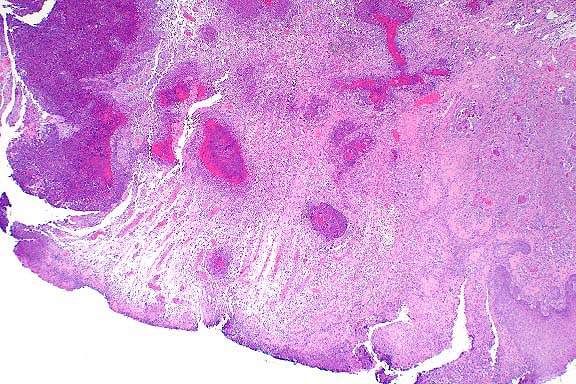The image appears to be a digitally created piece characterized by a blend of vivid colors and abstract shapes. Dominated by different shades of purple, pink, and white, the composition includes jagged fragments and irregular, curving forms that give it an almost topographical feel. The left side is marked by clusters of darker purple, punctuated with circular areas of even deeper hues, while lighter pink and white crack-like lines scatter across the right side, culminating in a more granular, sandy texture. The background is starkly white, serving as a blank canvas that accentuates the colorful, random spread of the image. The lack of any textual context or definitive imagery lends it an enigmatic quality, making it resemble a thermal satellite image, a painting, or even a mishap like a liquid spill, inviting multiple interpretations while hinting at a snowy landscape through its scattered white regions.